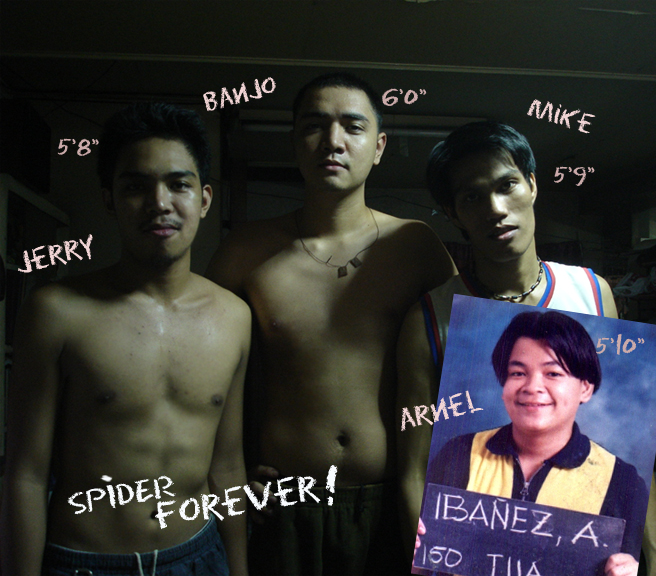In this image, we see three young Asian men positioned at the center, standing against a dimly lit indoor setting that resembles a gymnasium. The man on the left, identified as Jerry, stands shirtless, marked with the text "Jerry 5 feet 8 inches." The man in the middle, Banjo, is also shirtless, standing at "6 feet" and wearing a necklace with two small squares. On the right, Mike stands at "5 foot 9," donned in an Oklahoma City jersey. Mike holds a photograph depicting two individuals. This photograph is located in the bottom right corner of the image and shows another young man named Arnell. Arnell is attired in a blue shirt with yellow detailing along the shoulders and chest, and the partial text visible reads "I-B-A-N-E-Z comma A." Other written elements in the image include the phrase "R and L five foot ten a spider forever." The dominant colors in this image are black, white, tan, blue, red, yellow, and gray. The juxtaposition of the shirtless men and the additional photo they hold creates a multifaceted and detailed scene.